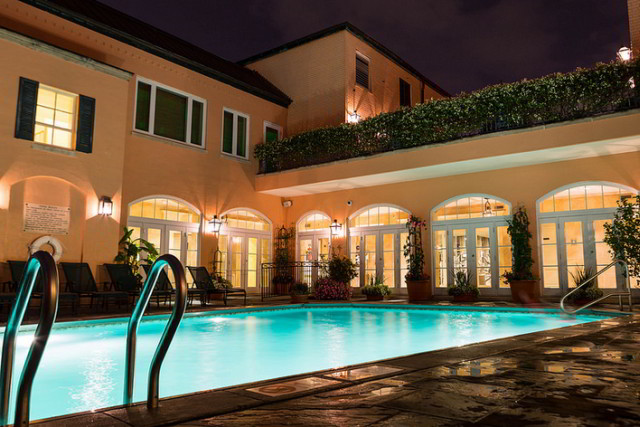The image depicts a beautifully illuminated outdoor scene at night, showcasing what appears to be a hotel with a striking resemblance to a lavish private residence. The setting features a rectangular, blue-lit swimming pool that extends diagonally from the lower left corner towards the center right. The pool is bordered by wet flagstone pavement and equipped with two stainless steel ladders for easy entry and exit. On the far side of the pool, there are five lounge chairs arranged in a row, complemented by potted plants scattered around the pool's edge. A life preserver is visible to the left.

In the background, a gorgeous tan or pinkish stucco building stands majestically, rising two and a half to four stories high. The building facade is adorned with multiple French doors and arched windows, all illuminated from within, indicating a welcoming warmth. The lower level features roughly six sets of glass doors, while the upper levels are mostly dark except for a few lit windows. On the second level, there is a balcony with hedges, adding a touch of greenery to the scene. The roofline is varied, with sections appearing slanted and tiled in black. An elegant series of lantern-like outdoor lights enhances the nostalgic ambiance, and various architectural details, such as drainpipes and ornate balconies, contribute to the building's distinguished appearance. Overall, the picture captures an enchanting, serene atmosphere under a starlit sky, devoid of people but rich in visual appeal.